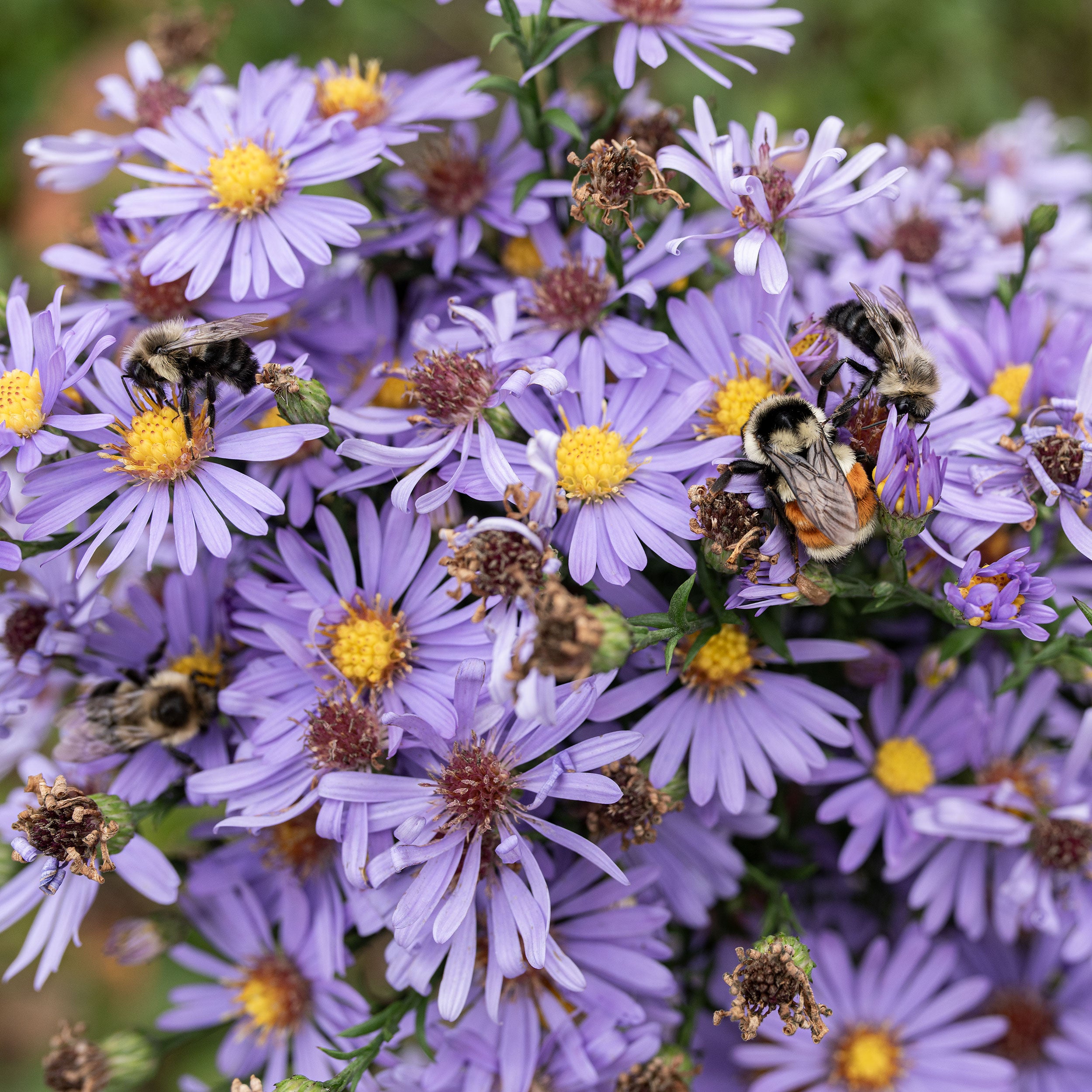This photograph features a vibrant, close-up view of a large cluster of flowers that resemble daisies. The petals of these flowers are a striking, light purple, and the centers are a bright, vivid yellow. The scene is teeming with life as several bumblebees—furry and about half an inch long—can be seen pollinating the flowers. Some of the flowers have fully bloomed, showcasing their radiant colors in sharp detail, while others are in various stages of wilting, with petals either fallen or turning brown. The greenery that mingles with the flowers and forms the blurred background adds depth to the outdoor setting, emphasizing that this is likely in a garden. The intricate details of the petals, the dynamic presence of the bees, and the natural setting make this image a captivating snapshot of nature's beauty and activity.